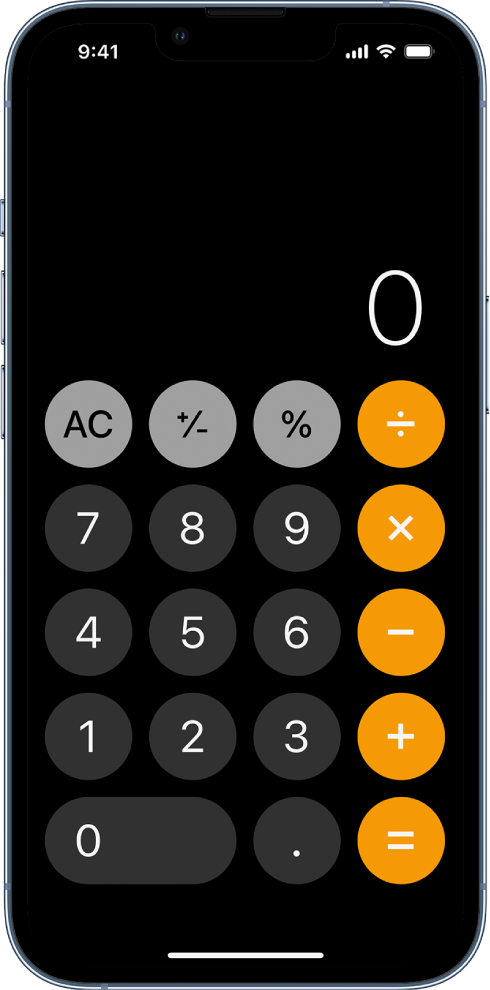This image depicts the screen of a powered-on cell phone displaying a calculator application against a black background. In the top left corner of the screen, white text displays the time as 9:41. The top right corner features icons indicating a strong cellular connection, a robust wireless signal, and a battery that appears to be nearly or completely full.

Below the status bar, taking up most of the screen, is the calculator interface. On the right side of this interface, a large white zero is prominently displayed, signifying that no calculations have been entered yet.

The calculator itself is organized into clearly defined rows and columns of buttons, each contained within a circular background. The first row comprises four buttons: an "AC" button within a circle, followed by a circle with a "±" symbol, then a circle with a "%" sign, and finally, a circle with an orange background featuring a division symbol.

The second row includes buttons for the numbers seven, eight, and nine in gray circles, followed by a button with an orange background and the multiplication ("×") symbol. The third row contains buttons for the numbers four, five, and six in gray circles, followed by an orange-background button with the subtraction ("−") sign. 

In the fourth row, buttons for the numbers one, two, and three are aligned in gray circles, while an orange circle contains an addition ("+") symbol. The final row features a wide gray circle for the number zero, a small gray circle for the decimal point ("."), and an orange circle for the equals ("=") sign.

The calculator layout is simple yet functional, adhering to a color scheme that uses gray for most of the number buttons and orange for the main operational symbols, providing clear visual distinctions for usability.